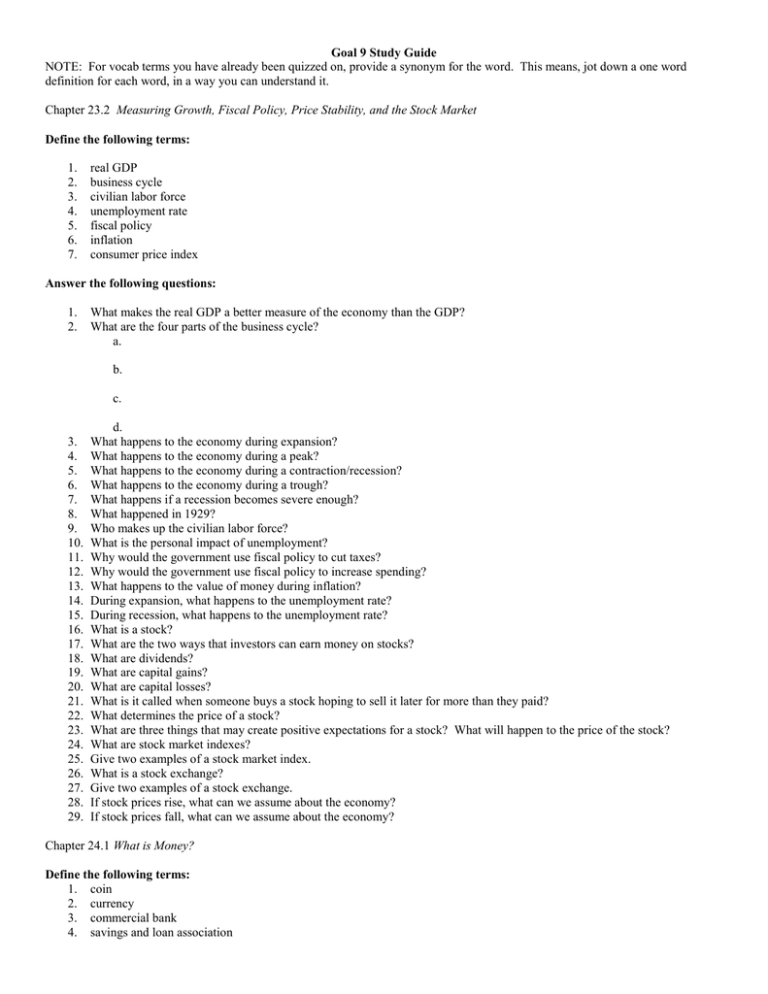A typed study guide titled "Goal 9 Study Guide" with detailed content on GDP, business terminology, and fiscal policy. The document includes a section labeled "NOTES" in all caps, providing terminology and instructions to write synonyms for previously quizzed vocab terms. It focuses on chapter 23.2, covering topics such as measuring growth, fiscal policy, price stability, and the stock market. Bold headers prompt definitions for key terms like real GDP, business cycle, civilian labor force, unemployment, fiscal policy, inflation, and the consumer price index. Following this, there are 29 comprehensive questions, beginning with the comparative advantages of real GDP over nominal GDP, covering detailed aspects of the business cycle, and discussing the factors influencing stock prices. The guide concludes with a bolded section to define additional financial terms: coin, currency, commercial bank, and savings and loan association. This study guide, typed in black and white, is presumably for a classroom setting aimed at helping students prepare thoroughly for an upcoming test on these economic principles.